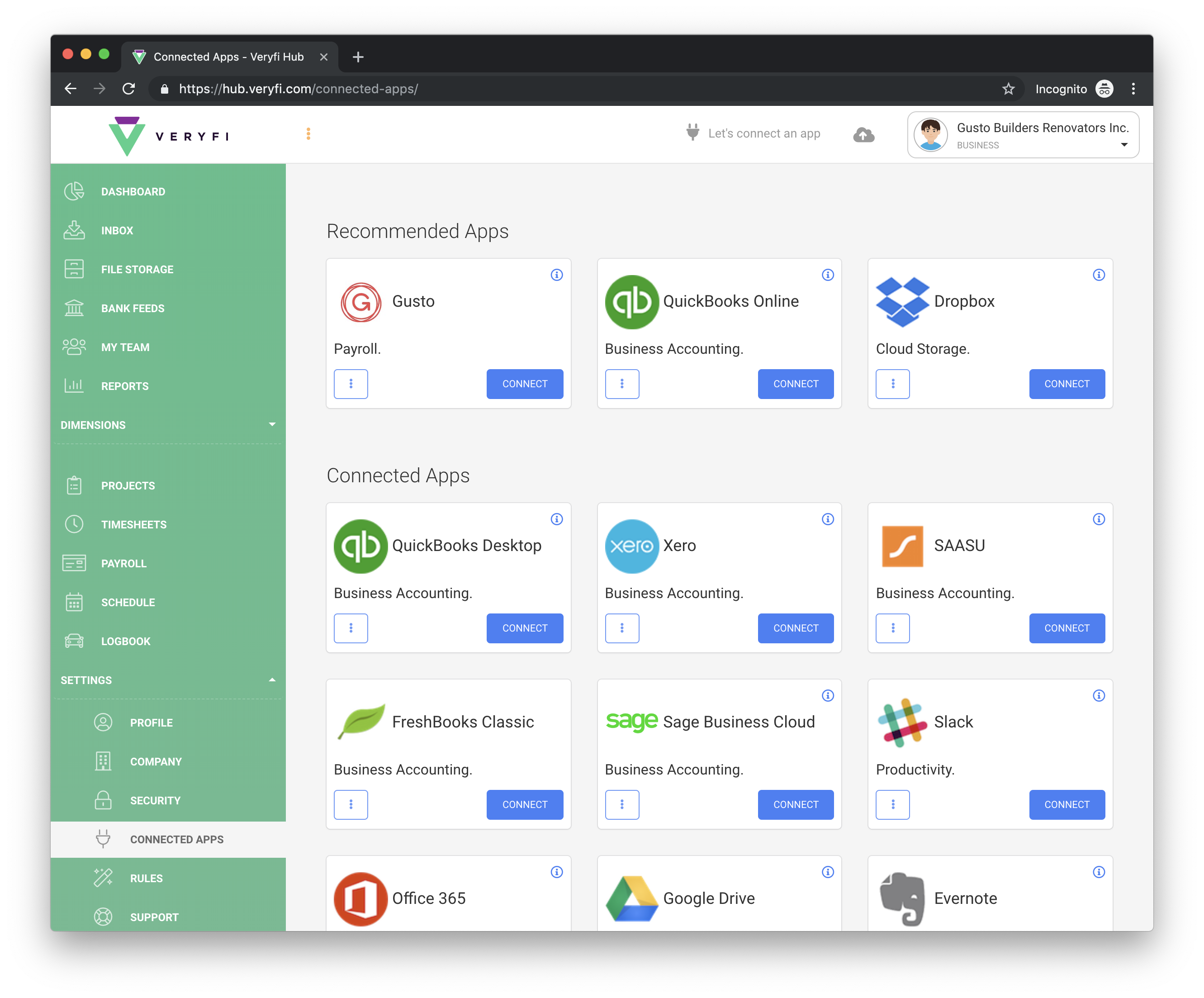This image is a detailed screen capture of a computer monitor displaying the "Connected Apps Verify Hub" webpage in an incognito browser window. 

At the very top, a dark gray bar features three circular buttons in the upper left-hand corner: red, yellow, and green, respectively. Positioned within this bar is a green V-shaped logo followed by the text "Connected Apps Verify Hub," indicating the name of the active tab. 

Directly beneath this bar, the incognito status and the secure connection to the site "hub.verify.com/connected-apps/" are clearly indicated, ensuring privacy and security. Below this, a white navigation bar showcases the green V-shaped "verify" logo on the left, flanked by the action options "Let's connect an app" represented by a plug icon, and a cloud icon with a white up-arrow indicating an upload feature. 

On the far right, the user's profile details are visible, mentioning "Gusto Builders Renovators Incorporated Business" with a cartoon icon depicting a young man with dark hair beside it.

A dark green vertical banner runs along the left side of the screen, listing various navigational options in white text: Dashboard, Inbox, File Storage, Bank Feeds, My Team, Reports, Projects, Timesheets, Payroll, Schedule, Logbook, Profile, Company, Security, Connected Apps, Rules, and Support. The "Connected Apps" option is highlighted, indicating the current selection.

The main section of the screen consists of two parts. At the top, under the header "Recommended Apps," suggested applications including Gusto, QuickBooks Online, and Dropbox are displayed. Below this section, under "Connected Apps," a series of linked applications are shown in a grid format: QuickBooks Desktop, Xero, Sasu, FreshBooks Classic, Sage Business Cloud, Slack, Office 365, Google Drive, and Evernote.

The image offers a comprehensive overview of the user interface, highlighting its segmented, user-friendly design and the variety of integrated applications available for business use.